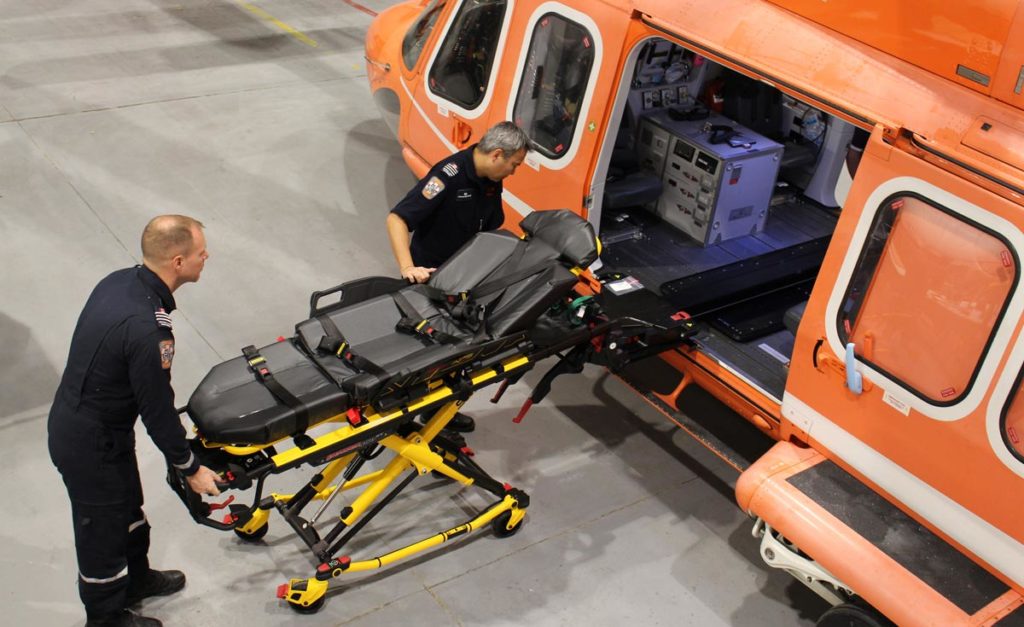In the image, a paramedic team is engaged in an air rescue operation. The scene is set inside a hangar with a concrete or asphalt-grey floor, casting numerous shadows. A bright red helicopter, accented with white around its window frames and filled with various panels, equipment, and controls, is stationed centrally towards the top right. Two men, both wearing black jumpsuits, are meticulously maneuvering a stretcher into the helicopter. The stretcher features a black bed with a yellow frame, along with several black and red components. One man with gray hair is positioned centrally, while the other, slightly balding, stands closer to the bottom left corner. They collaboratively guide the stretcher towards the helicopter, emphasizing the coordinated effort in this paramedic rescue scenario. The color palette of the scene includes striking shades of orange, cream, black, yellow, tan, beige, gray, and green, contributing to the detailed and dynamic visual description.